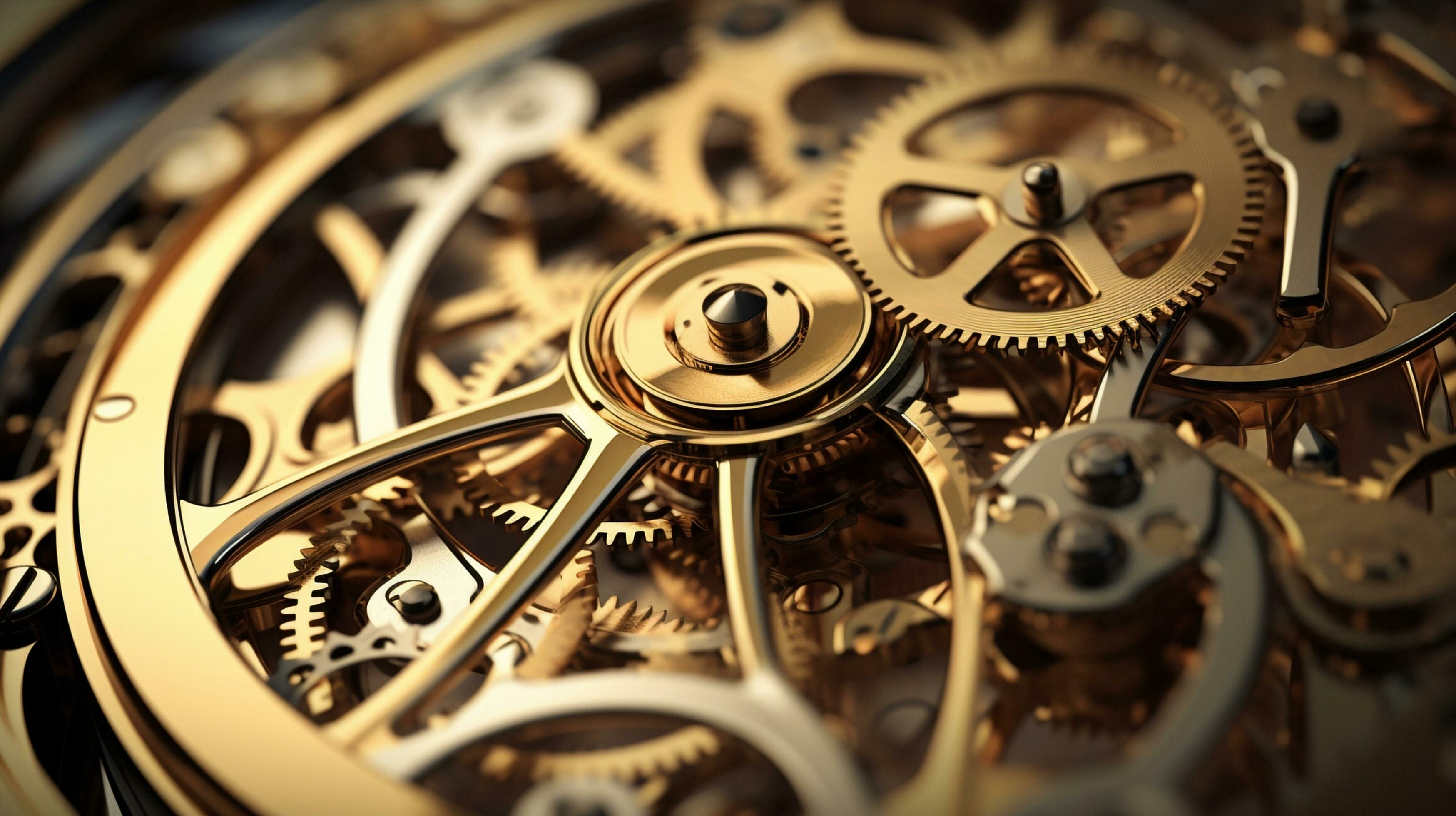This detailed close-up image showcases the intricate inner workings of a traditional mechanical watch. Predominantly featuring a composition of gold and brass metals with a hint of silver, the image captures an array of interconnected gears, delicate springs, and bolts. The circular formation of these components highlights their technical sophistication, with visible jagged-edged pieces likely contributing to the watch's mechanism. The exquisite craftsmanship suggests a high-value, shiny, and luxurious appearance. This meticulously detailed view emphasizes the precision required for such a timepiece, where even the slightest misalignment of parts could impair its function, underscoring its technical and delicate nature. This image is a testament to the craftsmanship of old-fashioned, wind-up watches, far removed from modern smartwatches, and encapsulates the timeless elegance of classic horology.